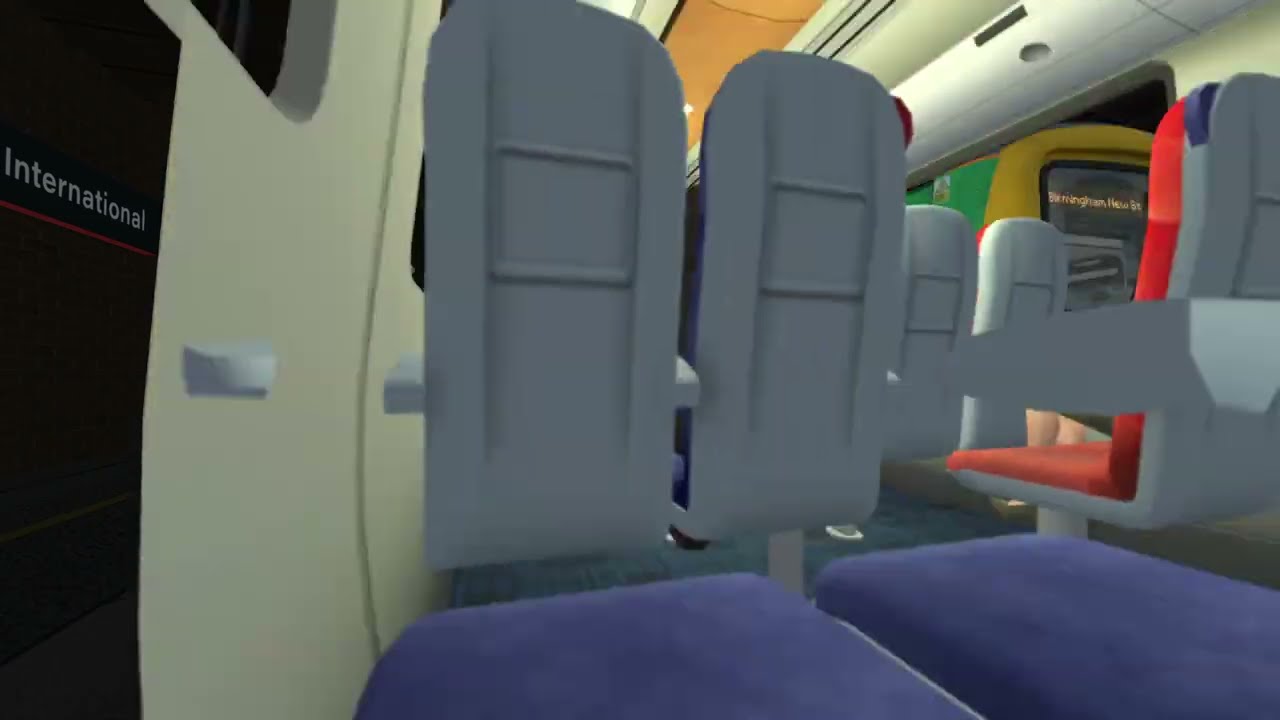This is a screenshot from a video game depicting the interior of what appears to be an aircraft cabin. The scene showcases a section of the cabin with a variety of seating arrangements and distinctive color palettes. On the left side, the wall is predominantly white, featuring a black window with the word "international" displayed in white lettering, underlined in red on a black rectangular area just below it. There are blue seats with blue cushions and gray backs that appear slightly separated from the seating portion. These seats are positioned in front of an aisle.

To the right, the aisle separates additional seats which face the opposite direction. These seats feature bright red cushions on both the bottom and back, complemented by gray armrests. In front of the red seats, there is a wall adorned with yellowish trim. This trim frames a rectangular screen displaying unreadable words, set against a tannish background. Above the seats on the right side, overhead bins and another messaging screen are visible. The roof of the cabin is white, traversed by a yellow stripe down the middle. The overall depiction suggests a computer-generated image, characteristic of a video game’s detailed rendering of an aircraft's interior.